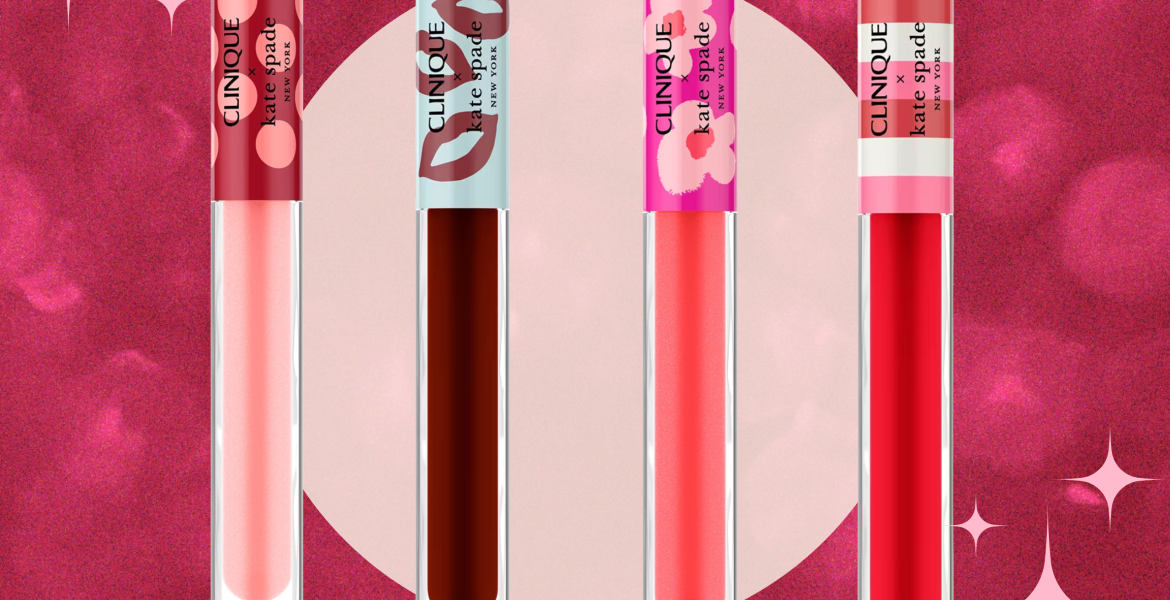The advertisement image features four distinctive cylindrical makeup products prominently aligned in front of a vibrant, raspberry-colored background with swirling lighter pink splotches and a partially cut-off large pink circle in the center. At the bottom right corner, pink diamond-like sparkles add a touch of glitter, with additional but partially cut-off pink stars visible at the top left. These makeup products, labeled "Clinique X Kate Spade, New York," likely represent lipsticks or lip glosses, given their vivid color schemes. The first item on the left is pink with a red label adorned with pink polka dots; the second is dark maroon with a white label featuring multiple kiss marks; the third is peach with a hot pink label decorated with pink flowers having red centers; and the last one is vibrant red with striped pink, white, and maroon lines. The image is purposefully designed to highlight the variety of shades and playful packaging of this collaborative beauty product line.